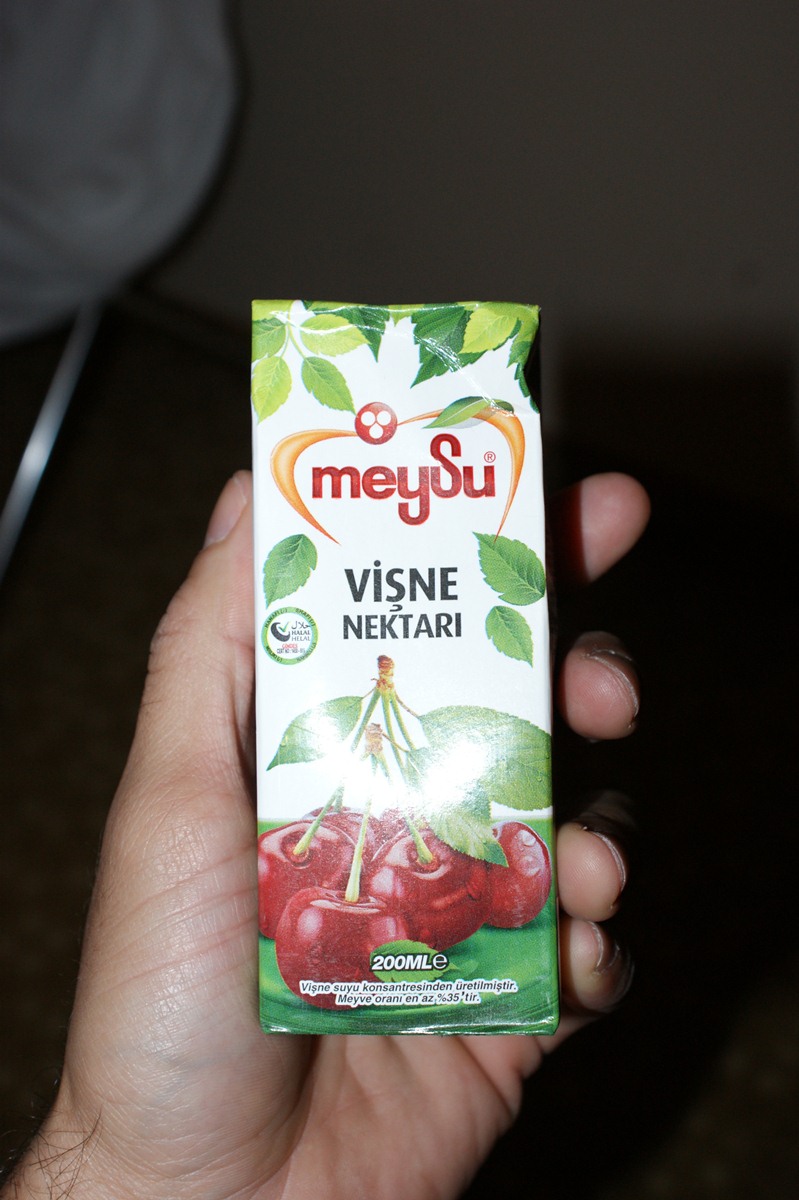In the portrait-oriented photograph, a person's left hand is prominently displayed against a dark background, possibly an appliance or tabletop. The hand's thumb is upright, pressed against the side of a juice box, while the four fingers wrap around its back showing the trimmed fingertips. The juice box, small and fitting comfortably within the hand, is primarily white with festive illustrations of variously colored leaves—dark green, light green, and almost yellow. The brand name 'Meysu' appears in distinct red lettering at the top, followed by 'Visne Nektari' in black letters, indicating it is a cherry-flavored nectar. At the bottom of the box, there's a vivid depiction of four to six glossy red cherries with green stems and leaves. Though the font is too small to read precisely, it mentions a 200-milliliter capacity along with other textual elements and icons that are not entirely legible due to their size.